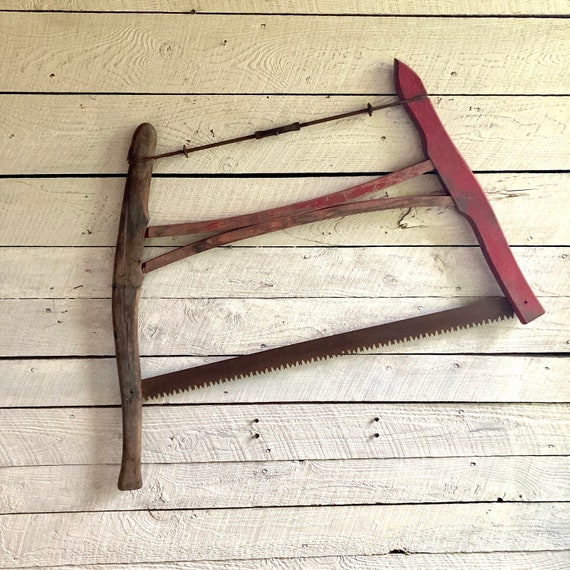The image depicts an old, handmade two-person saw, likely from the 1800s, resting on a surface of beige, creamy white, or light yellow wooden boards resembling deck material. The saw features a distinctive H-shaped frame, formed by a wooden handle on the left side and a red wooden piece on the right, connected at the top by a leather rope or metal wire. The horizontal bar in the middle, made of wood, links the two vertical wooden pieces. At the bottom, a rusted saw blade connects the structure. The background showcases unevenly painted wooden boards, indicating it's either a deck or perhaps siding of a house, with visible gaps and protruding nails.